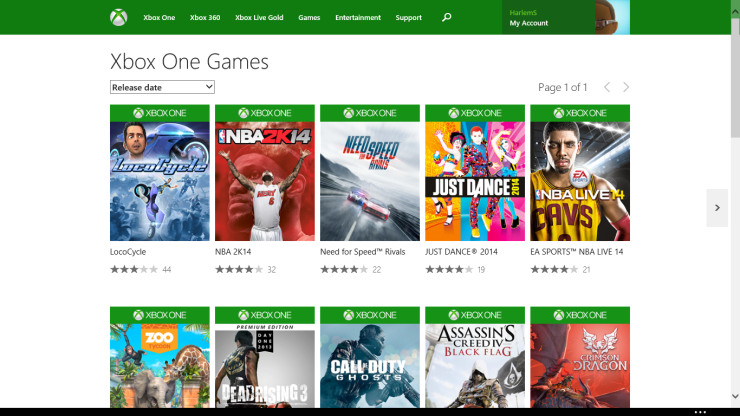Caption: 

A vintage screenshot of the Xbox website features an array of Xbox One games, reflecting its earlier state. The user, identifiable by the profile name "Harlem5," and an avatar snapshot featuring silver-framed glasses with brown-tinted lenses, seems to be browsing the selection. The games are displayed in two rows. The first row, from left to right, showcases *LocoCycle*, *NBA 2K14*, *Need for Speed Rivals*, *Just Dance 2014*, and *EA Sports NBA Live 14*. The second row, although partially obscured, hints at titles including a zoo-themed game, *Dead Rising 3*, *Call of Duty Ghosts*, *Assassin's Creed Black Flag*, and *Crimson Dragon*. Notably, *LocoCycle*, despite having the most reviews, has garnered a rating of only 3 out of 5.